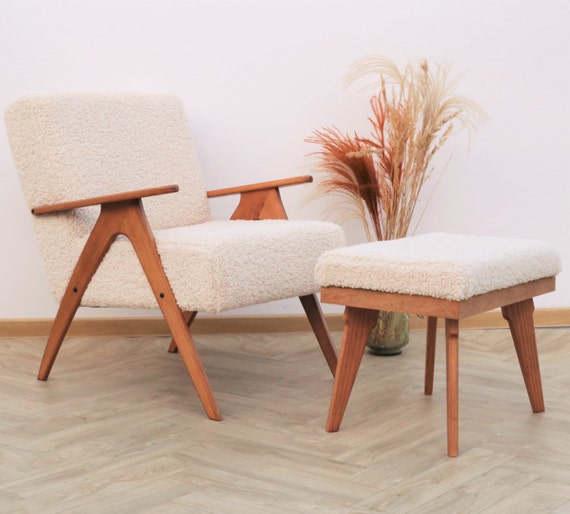This photograph, taken indoors with a soft, grayish tone and not very well-focused lighting, showcases a cozy seating arrangement centered around a fuzzy chair and a matching ottoman. Both pieces have a brown wooden frame, including smooth, round armrests and legs. The chair, positioned on the left, features a distinct design with the armrests curving down in an upside-down V-shape and housing two off-white, fluffy, cotton-like cushion squares that exude softness. The ottoman mirrors this style with a cushion that matches the chair's material, square in shape and equally cushy. 

The setup rests on a light beige wooden floor adorned with triangle-shaped designs. The surrounding environment includes white walls with a light brown baseboard along the bottom. A rectangular design is present on the floor, adding a subtle decorative touch. Behind the chair, there's a clear vase filled with decorative white and red grasses, enhancing the room's aesthetic. In addition, a pot with a plant can be seen, further complementing the scene. Overall, this image showcases a plush, inviting nook perfect for relaxation.